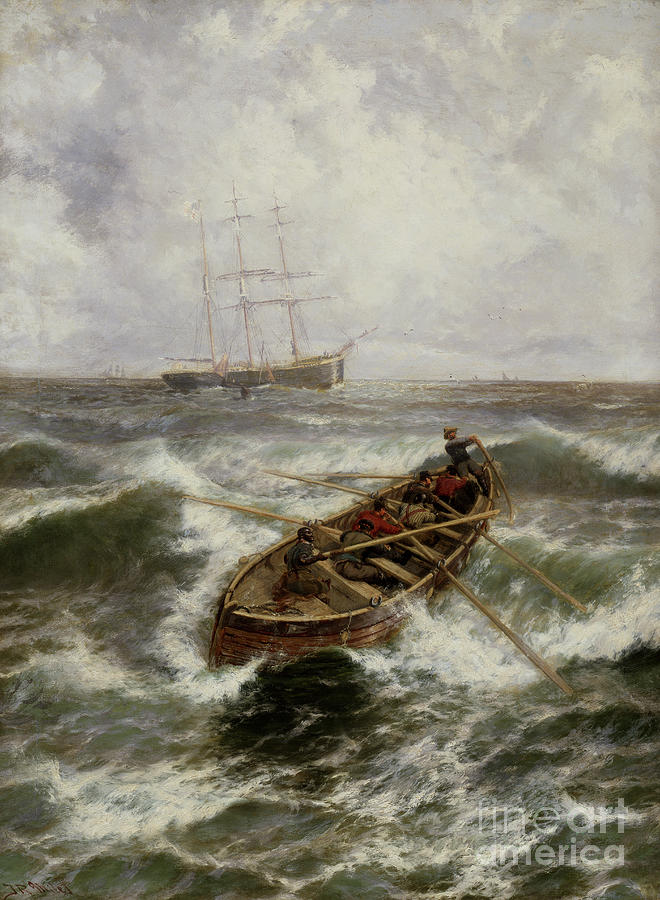This painting, rendered in portrait layout, captures a tumultuous ocean scene marked by stormy weather. The upper 45% of the canvas features a cloudy, predominantly blue sky, while the bottom 55% is dominated by rough, greenish-gray waters with tall, crashing waves. The primary focus of the artwork is a large, wooden rowboat being violently tossed by the waves. Positioned in the lower center of the canvas, the rowboat is manned by a group of men, some wearing red jackets, struggling to navigate through the fierce sea with oars in hand; one man stands at the bow, possibly directing their efforts. Scattered among them are various bags. In the background, closer to the horizon where the water meets the sky, a large, blue clipper ship with three towering masts is visible. Further back, another vessel with similar masts can be faintly seen through the thick gray clouds. At the bottom right of the painting, the text "FINE ART America" appears in white letters, subtly embedded within the scene.